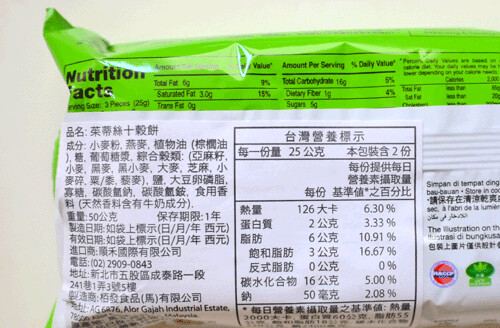This image displays the back of a small plastic package, oriented horizontally. The upper section of the package is lime green, prominently featuring a standard "Nutrition Facts" label that details the amounts of fat, fiber, sodium, sugars, and other nutritional information. The lower part of the package has a white label with black or dark brown text composed of Eastern characters, indicating that the package might be from an East Asian country. Although the exact details cannot be read, the layout suggests that the ingredients are listed on the left and a Nutrition Facts chart, similar to the one seen in America complete with percentage values, is located in the center. This arrangement provides essential nutritional details in both English and an Eastern language.